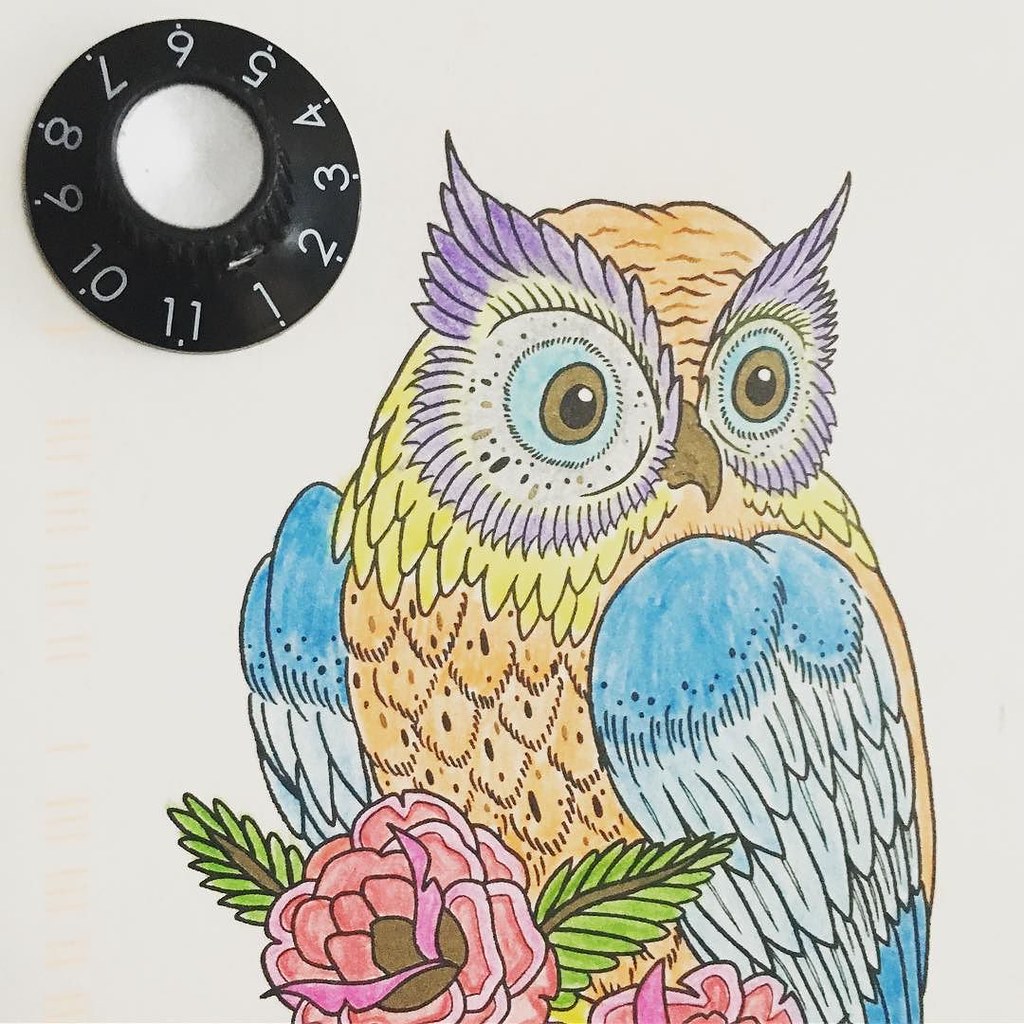A colorful illustration of an owl, presumably colored with pencils, is presented on a white coloring paper. The owl features vibrant blue and brown eyes, surrounded by purple feathers, an orange forehead, and yellow cheeks. Its chest and back are adorned in orange, while its wings showcase a mix of dark blue and light blue hues. The owl's beak matches the golden brown tone of its eyes. It is nestled among two flowers, each with pink and magenta petals and green leaves extending from both the top and side. In the upper left corner, there is a distinct black ring marked with white numbers from 1 to 11, resembling a dial without any hands or indicators. This detailed and vivid scene highlights the imaginative use of colors and careful attention to detail.